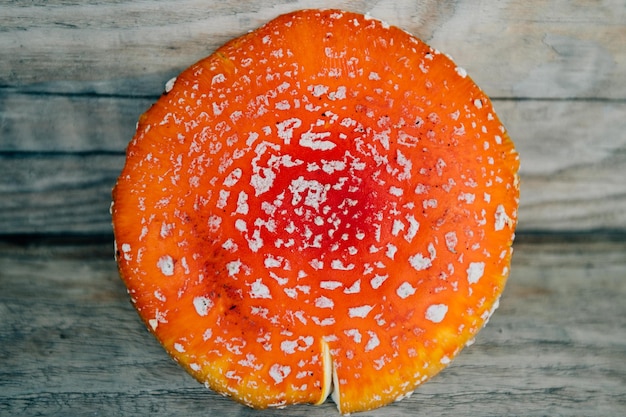A vividly colored circular object, likely a mushroom cap or possibly a fruit, sits prominently in the center of a weathered, gray-stained picnic table. This close-up image reveals intricate details: the object has a striking bright orange top that fades into yellow towards the edges, and a hint of dark red at the center. The surface is dotted with irregular white patches arranged somewhat symmetrically. The wooden table beneath, with its rough texture and visible grains, provides a contrasting background that enhances the vivid colors of the object. The cap or fruit appears to be sliced or has a natural cut on one side, exposing a whitish interior. This image, devoid of any text, captures the raw and natural beauty of the subject in an otherwise subdued setting.